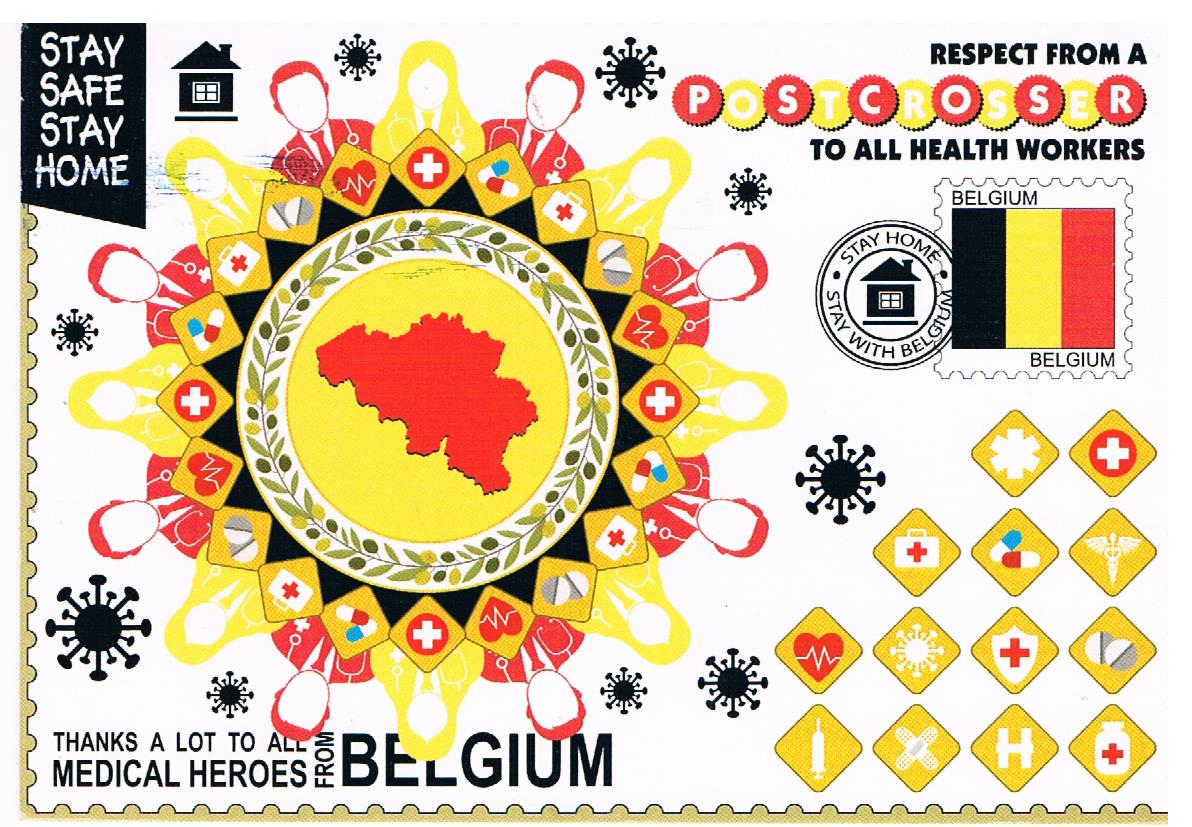This poster, likely created during the COVID-19 pandemic in Belgium, features a white background adorned with numerous elements in red, yellow, and black. Dominating the top right corner are bold black letters spelling "Respect From Postcrossers to All Health Workers," with the word "Postcrossers" alternating in red and yellow circles for each letter. Below this, there's a Belgian stamp depicted in black letters with the vertical stripes of the Belgian flag in black, yellow, and red next to it, accompanied by a round stamp inscribed with "Stay Home, Stay With Belgium."

In the center, a yellow map of Belgium, outlined and filled in red, is encircled by various medical icons and symbols, such as crosses, pills, a medical table, a heart with a heart rate, and a red cross sign. Surrounding these symbols, there are stylized outlines of men and women believed to represent healthcare workers. Interspersed around these figures are icons representing the COVID-19 virus with its distinctive spiked structure.

To the upper left corner of the poster, there's another rectangular section with the phrase "Stay Safe, Stay Home" in white letters. 

At the bottom of the poster, the message "Thanks A Lot To Our Medical Heroes From Belgium" is prominently displayed in black print. In the lower right corner, additional medical icons recur, featuring a heart, an injection syringe, a Band-Aid, and the COVID virus icon.

Overall, the poster vividly combines symbolic imagery and heartfelt messages to honor and encourage healthcare workers during the pandemic in Belgium.